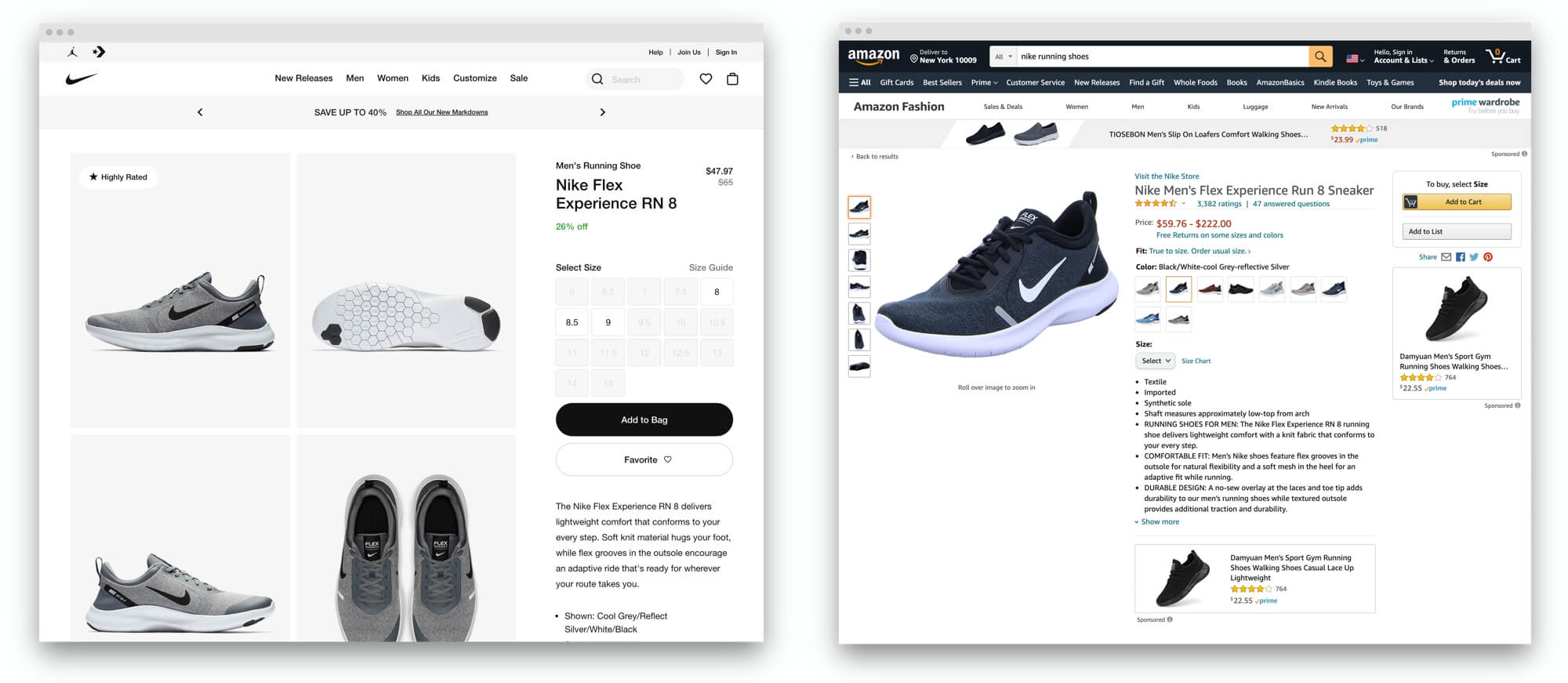**Detailed Caption for Image Comparison of Two Ads:**

The image displays two distinct advertisements side by side.

**Right Advertisement: Amazon Prime Ad**
On the right, the Amazon Prime ad has a compact, square design with a predominantly black background adorned with white and yellow text. The top-left corner prominently features the Amazon logo, consisting of the word "Amazon" in white followed by a yellow arrow underneath, suggesting a smile. Below the logo, it reads "Deliver to New York 10099".

A substantial part of the ad is dedicated to a search bar, highlighted in white, indicating a search for "Nike running shoes". Adjacent to the search bar is a yellow button featuring a black search icon. Also on this line are symbols and text like a small USA flag, "Hello, Sign in", "Accounts & Lists", "Returns & Orders", and a shopping cart showing "0" items in yellow.

Underneath, there's a navigation bar with various links in white text, such as "All", "Gift Cards", "Bestsellers", "Prime", "Customer Service", "New Releases", "Find a Gift", "Whole Foods", "Books", "Amazon Basics", "Kindle Books", "Toys & Games", and a highlighted "Shop Today's Deals".

Further down, the ad showcases two pairs of shoes. The first shoe is labeled "Tyusfun Men's Slip-on Loafers Comfort Walking Shoes" priced at $23.99, marked with four gold stars and tagged as Prime eligible with 518 five-star reviews. The second shoe is "Nike Men's Flex Experience Run 8 Sneaker", with a link to visit the Nike store. This listing includes a rating of four and a half stars from 3,382 reviews, with a price range of $59.76 to $220.22. It also mentions "Free Returns on some sizes and colors", "True to size, order usual size", and details various color and size options. A highlighted product image showcases the shoe in black with a white sole, with a drop-down menu for selecting sizes and a size chart link.

At the bottom of the ad, another shoe's picture appears alongside its price and rating. A banner beneath these details provides buttons to "Add to Cart", "Add to List", and sharing options via email, Facebook, Twitter, and Pinterest.

**Left Advertisement: Alternate Nike Ad**
The left ad features a gray background, mainly showing the top headers like "New Releases", "Men", "Women", "Kids", "Customized", and "Sale". It includes a search bar, help link, and options to "Join Us" or "Sign In".

Prominently positioned, it advertises the "Nike Flex Experience RN8" running shoe for men, previously priced at $65, now $47.97, indicating a 26% discount in green text. Size options available are 8, 8.5, and 9. A white banner below provides a button to "Add to Bag" and a favorite option.

The ad also prominently displays four images of the shoe, depicting it in black and white. Text below the images gives a detailed description of the shoe.

**Summary:**
Both ads primarily focus on Nike running shoes, each offering detailed product descriptions, imagery, and various purchasing options. The Amazon Prime ad features a more comprehensive and interactive design with a wider array of navigation links and customer reviews, while the alternate ad on the left provides a straightforward, clean layout focused directly on the product's price, discount, and available sizes.